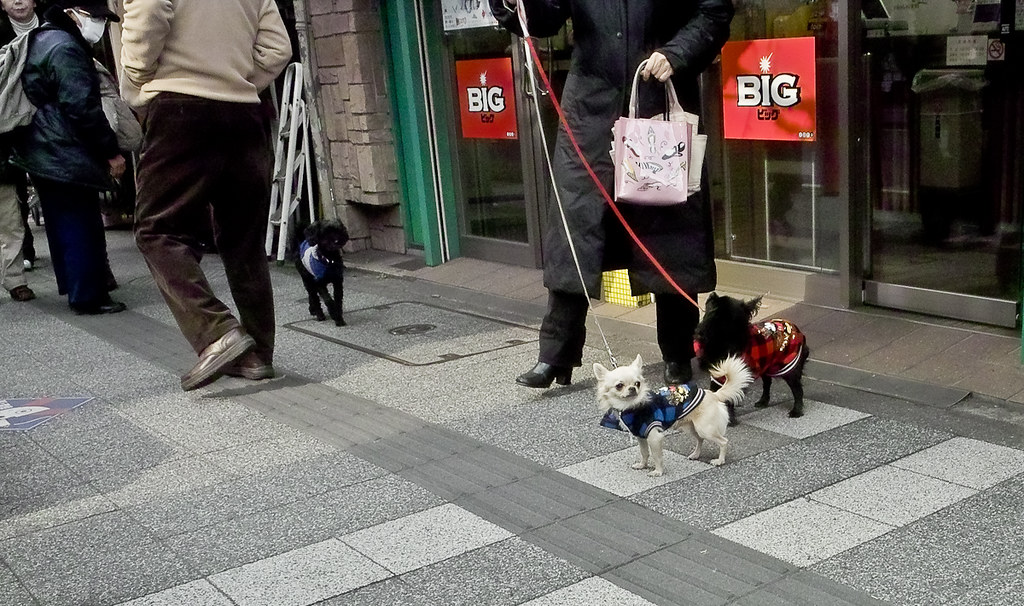A daytime photograph captures a lively street scene with multiple individuals walking on a tiled sidewalk composed of light and dark gray sections, including a dark gray tactile path in the center to prevent slipping. Prominently, there is a figure emerging from a store with glass front doors rimmed in green, holding a pink handbag in their right hand and two leashes in the left, one red and one white. The red leash attaches to a black fluffy dog dressed in a red plaid shirt, while the white leash secures a beige dog with tan accents in a blue jacket. Both dogs appear small, resembling Chihuahuas. Adjacent to them is a person in a white face mask, a dark blue or gray raincoat, blue trousers, and black shoes, observing the scene. Another individual, wearing a beige sweatshirt, black pants, and brown shoes with black soles, walks beside a black dog in a blue and white sweater. Additional figures include someone in a white turtleneck, black jacket, beige pants, and brown shoes, facing the camera, and another with a black jacket over a white undershirt. The framing cuts off the upper bodies of the individuals, focusing on their attire and the bustling activity on the sidewalk. In the distance, a black dog with a blue and white shirt walks independently. The setting also features a red square sign with white lettering "B.I.G." and text in a foreign language on the store's door.